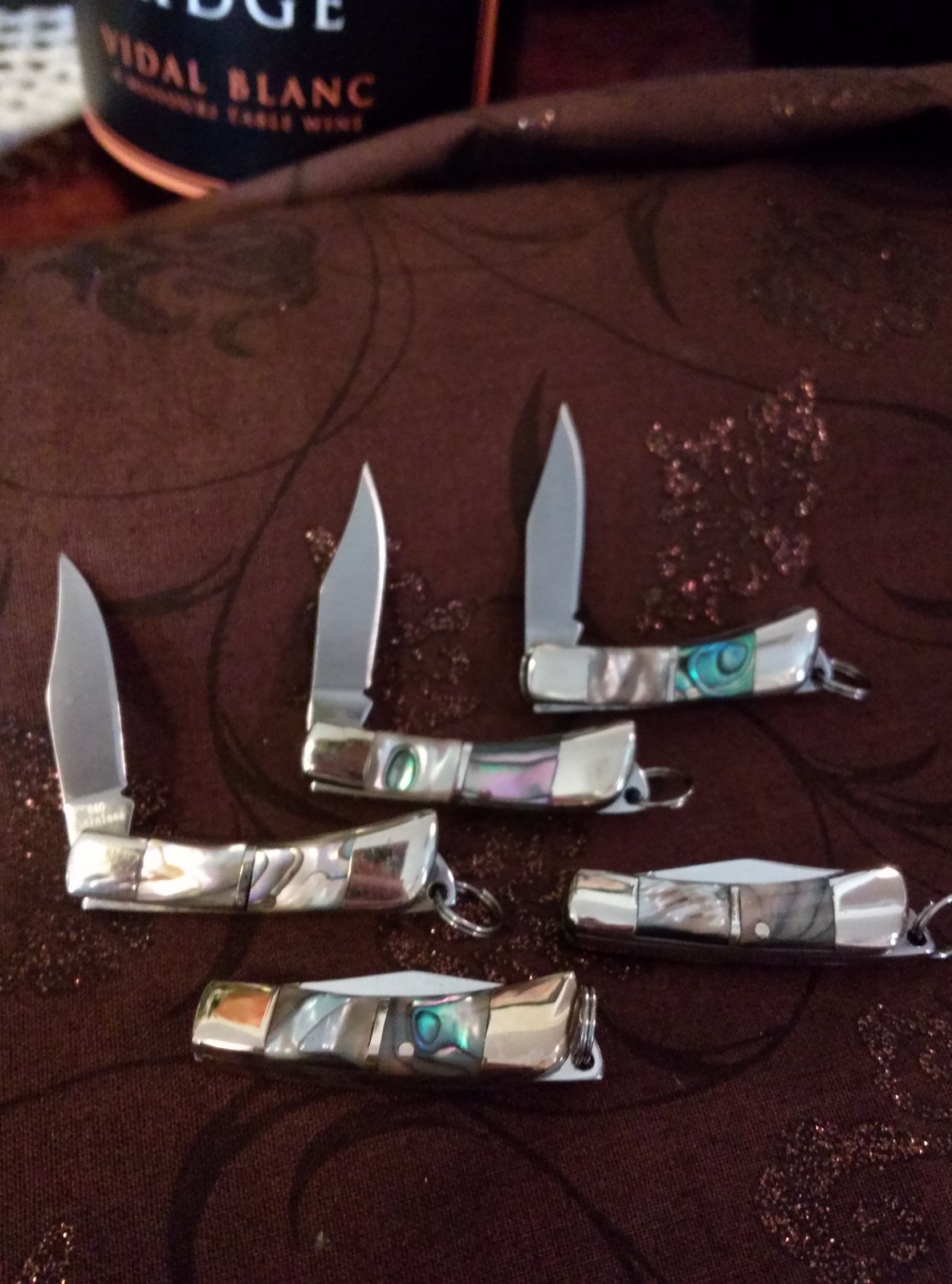This color photograph prominently features five flick knives placed on a rounded, brown tablecloth adorned with a floral pattern in a slightly darker hue, including long lines that might represent stems. Three of the knives are open, with their blades forming 90-degree angles, while the other two remain closed, showcasing only the triangular blade tips protruding from their handles. Each handle is distinctly designed with elaborate, multi-colored patterns, inlaid faux gems, and sections of pearlescent material, lending a unique and intricate appearance to each knife. Towards the left side of the image, partially out of focus, is the bottom of a wine bottle with a black label featuring the words "Vidal Blanc" in orange. This bottle, coupled with the detailed exoticness of the knives, adds an intriguing context to the scene captured on the maroon-colored cloth.